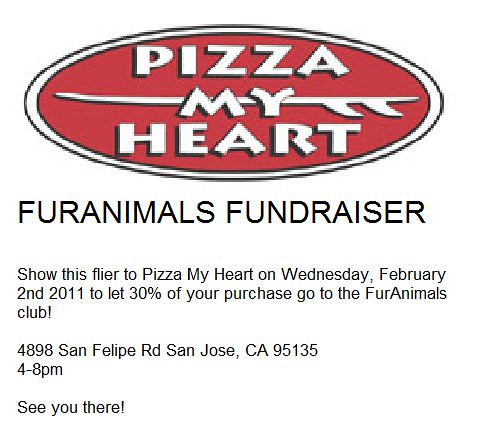This advertisement features a clean, white background with a distinct red, oval-shaped logo at the top, bordered in white and outlined with a thin black line. Inside the logo, in large, bold white block letters with black shading, are the words "PIZZA MY HEART," stacked vertically. An arrow-like symbol runs behind the word "MY." Below the logo, in prominent black all-caps, the text reads "FUR ANIMALS FUNDRAISER." Beneath that, in smaller, left-aligned font, are the details: "Show this flyer to Pizza My Heart on Wednesday, February 2, 2011, to let 30% of your purchase go to the Fur Animals Club." Following the event details are the location and time: "4898 San Felipe Road, San Jose, California 95135, 4 to 8 p.m." The flyer concludes with a friendly invitation, "See you there!"